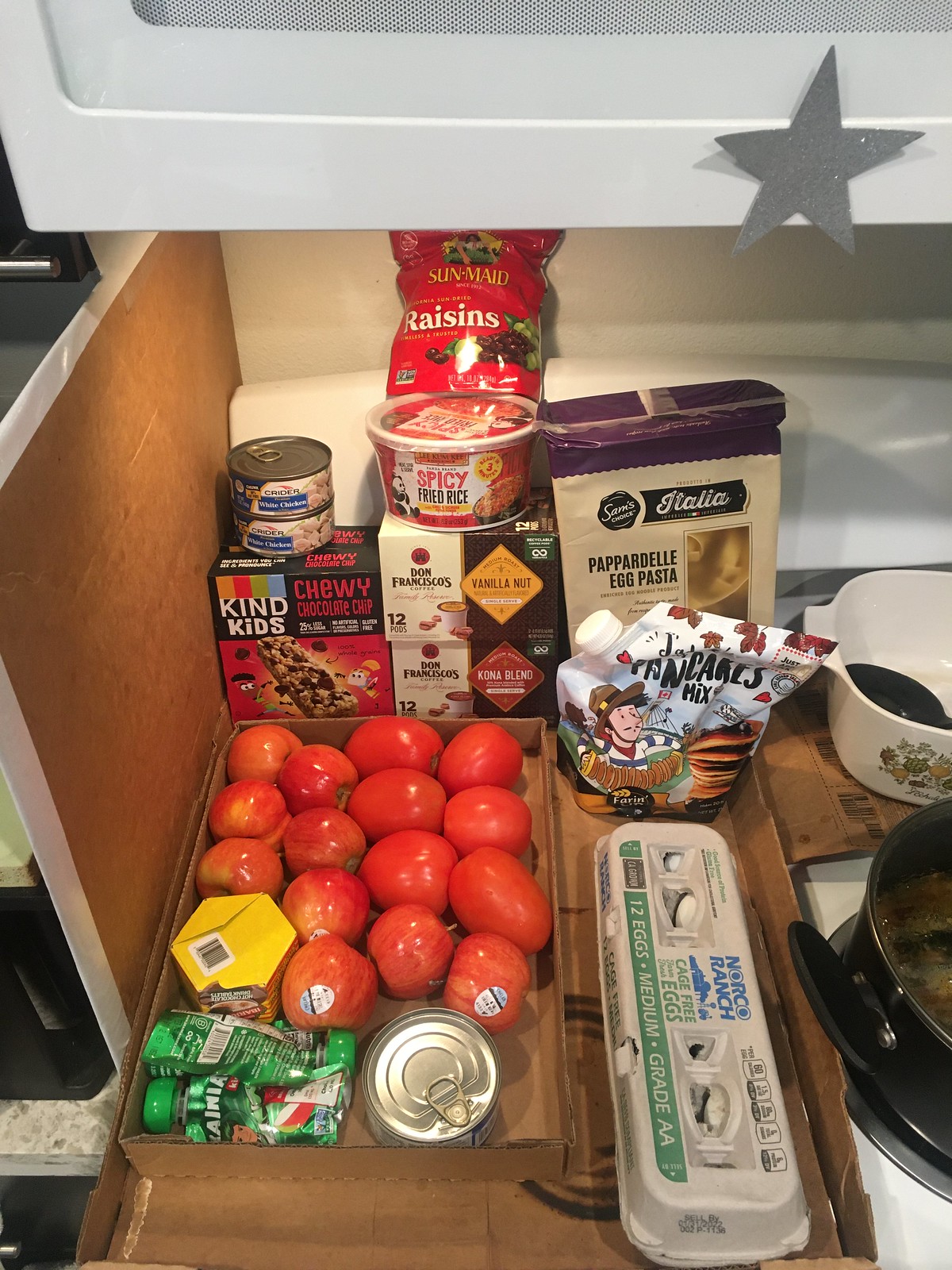This realistic photograph captures the scene of a bustling kitchen right after a recent grocery trip. On the right side, a range is actively in use with a black pot of water or broth boiling away, emitting light steam. Behind the black pot sits a white glass pot with a smaller black scoop nestled inside. 

To the left of the range, a long, flat cardboard box is filled with an array of recently purchased food items. In the bottom right corner of the box, a carton labeled "12 Eggs Medium Grade A" is visible. Directly above the eggs, a sack of pancake mix prominently displays an illustration of a cowboy along with a convenient pour spout. 

To the back of the box, a package of "Pappardelle Egg Pasta" with its contents visible through a window peaks out. Moving leftward, a box filled with cans of tomatoes can be seen, accompanied by a box of chewy chocolate chip granola bars and two boxes of coffee pods. Supplementing this assortment, there is also a container of spicy fried rice and a bag of raisins situated above the granola bars and the coffee pods. The composition of the kitchen setting and the variety of foods captured convey a sense of homely comfort and readiness for meal preparation.